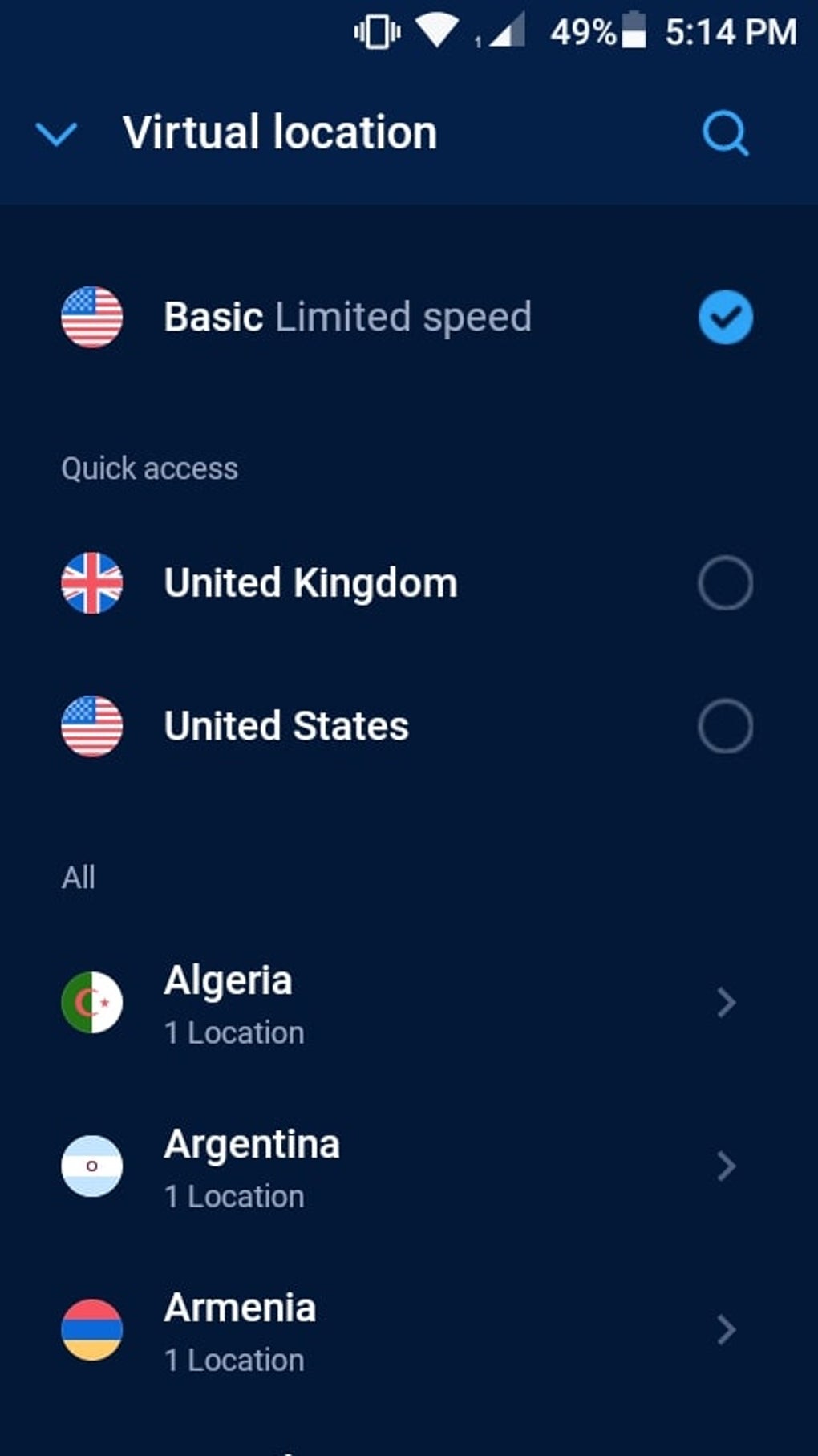The image showcases a user interface of a phone-based VPN app. At the top of the screen, there are several phone status icons including a vibrating phone symbol, network signal, Wi-Fi signal, phone network type, battery level which is at 49%, and the time displayed as 5:14 PM. Below these icons, a section labeled "Virtual Location" is visible, indicating various location options.

At the top of this section, the word "Basic" appears alongside a circular icon featuring the colors of the US flag. Next to this, the description "Limited Speed" is written in lighter letters, and a check mark indicates this option is selected.

Beneath this, there are two primary sections: "Quick Access" and "More Locations." In the "Quick Access" section, two options are indicated: United Kingdom and United States, both selectable. In the "More Locations" section, the app lists available locations including Algeria, Argentina, and Armenia, each noted with a single available location.